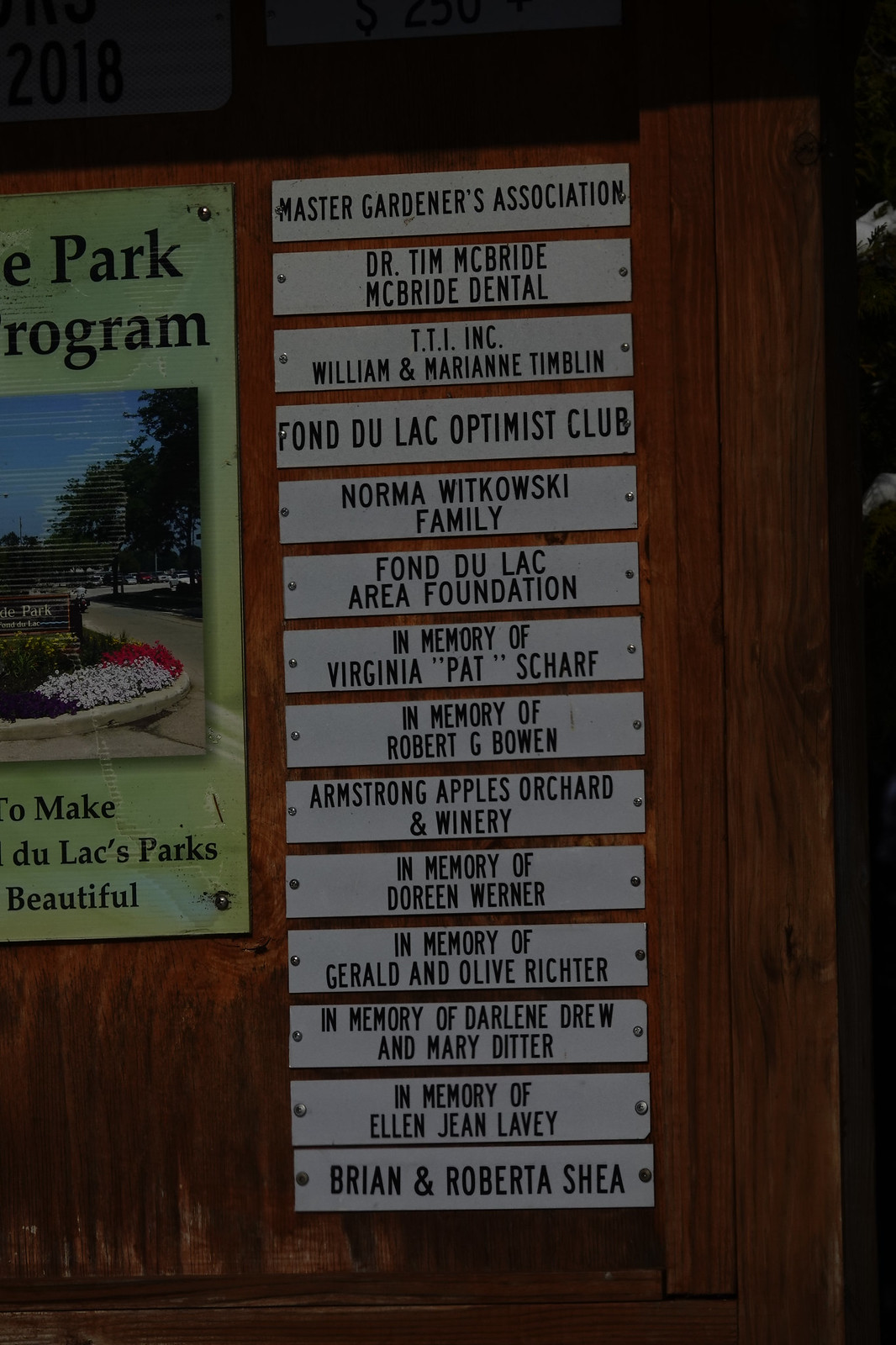This image features a vertically aligned, rectangular display against a wooden wall or door, with a somewhat dark setting suggesting it could be either indoors or outdoors. Dominating the center of the image is a wooden signboard with a series of metal plaques affixed to it, each bearing the names of various sponsors and memorial dedications. From top to bottom on the right side, the plaques read: "Master Gardeners Association," "Dr. Tim McBride, McBride Dental," "TTI Inc.," "William & Marianne Timbaland," "Fond du Lac Optimist Club," "Norma Witkowski Family," "Fond du Lac Area Foundation," "In Memory of Virginia Pat Scharf," "In Memory of Robert G. Bowen," "Armstrong Apples Orchard & Winery," "In Memory of Doreen Werner," "In Memory of Gerald & Olive Richter," "In Memory of Darlene Drew & Mary Ditter," "In Memory of Ellen Jean Lavi," and "Brian & Roberta Shia." Each of these names is centered on a white background with screws on either side, securing them to the wood. To the left, a partially visible larger sign with a green background and brown text features an image of flowers but is cut off by the edge of the photo, suggesting the continuation of the design beyond the frame. The overall setting, adorned with a mix of brown, white, black, green, and blue colors, appears to be a list of sponsors, possibly located in a park or a similar communal outdoor area.